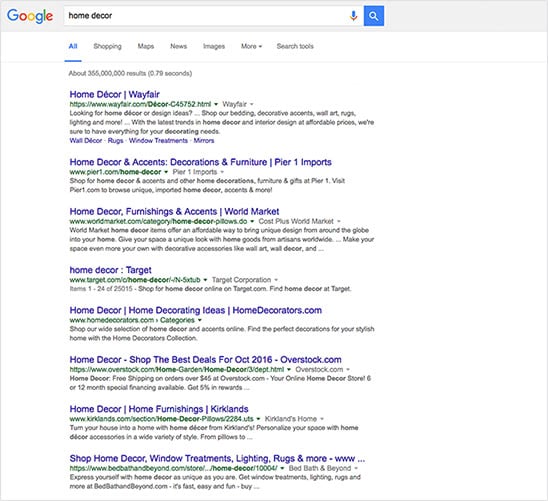The image is a screenshot of a Google search page in portrait orientation. The background is predominantly white, with a light gray horizontal bar running across the top. On the left side of this bar is the iconic Google logo, featuring a blue "G," a red "O," a yellow "O," a blue "G," a green "L," and a red "E." 

Below the logo, within a white search bar, the words "home decor" are typed in black font. To the right of the text in the search bar, there’s a microphone icon indicating voice search capabilities, followed by a blue box containing a white magnifying glass symbol, which is the button to initiate the search. 

Beneath the search bar, various categories for filtering search results are listed, including 'All,’ ‘Shopping,’ ‘Maps,’ ‘News,’ ‘Images,’ and ‘More,’ as well as search tools. In this image, the ‘All’ category is highlighted in blue with a thin blue underline.

Directly under the category filters, it states the number of search results: “About 355 million results (0.79 seconds).”

Displayed are the first few search results for "home decor," with each result consisting of a blue header, a green URL, and a brief description in black text. The search results include:

1. **Wayfair - Home Decor & Accents, Decorations, and Furniture**  
2. **Pier 1 Imports - Home Decor Furnishings and Accents**  
3. **World Market - Home Decor**  
4. **Target - Home Decor**  
5. **Home Decorating Ideas - HomeDecorators.com**  
6. **Overstock - Home Decor, The Best Deals for October 2016**  
7. **Kirkland's - Home Decor, Home Furnishings, Window Treatments, Lighting, Rugs, and More**

Each entry succinctly describes the type of home decor products available at these retailers or websites.